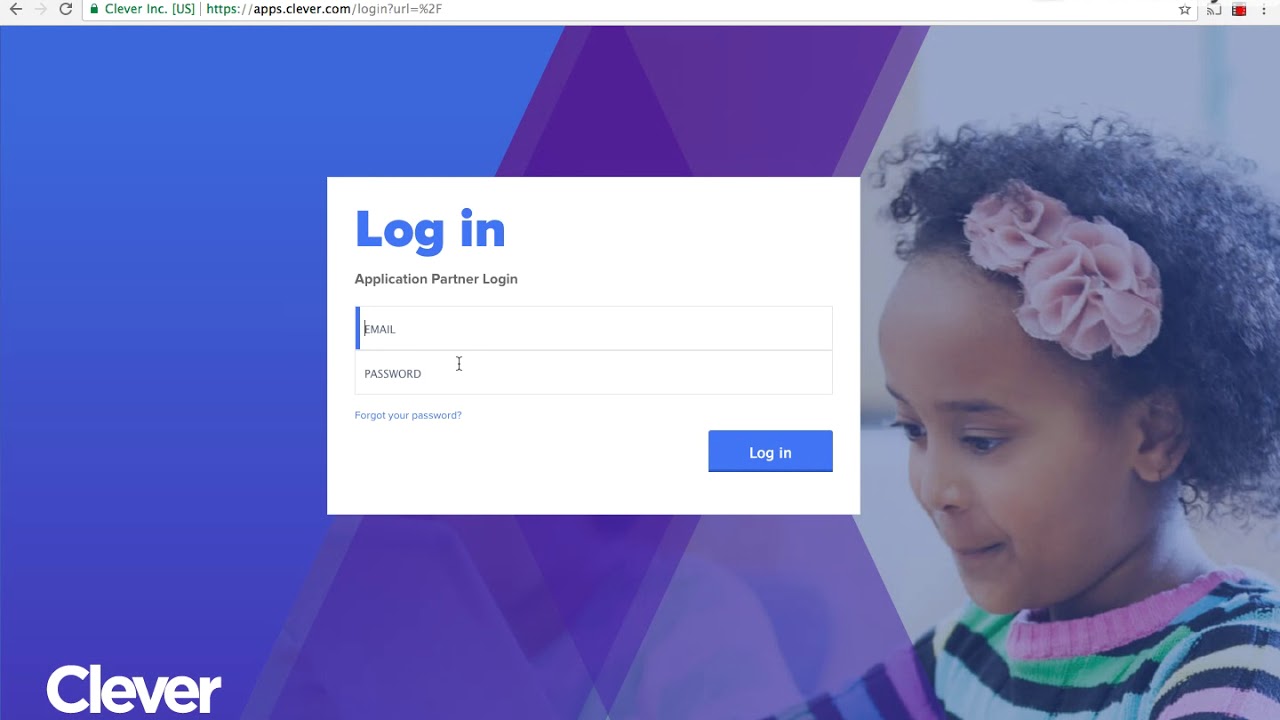The screenshot displays the login page of the website "Clever." The background of the page transitions from light blue on the left, to purple in the center, and finally to white on the right. On the right-hand side, there is a photograph of a young black girl who appears to be around eight or nine years old. She is smiling with her lips pursed and has a pink floral bow in her hair. She wears a knitted sweater with a pink collar and stripes in black, white, pink, blue, and lime green. Her eyes are cast downward, as if she is reading something.

At the bottom left corner of the page, the website’s name "Clever" is displayed in white letters. The login credentials section is centrally located within a white rectangle labeled "login" in bold blue font. Underneath this, in smaller black font, it reads "application partner login." There are two input boxes provided for entering an email address and a password. Below these fields, there is a blue link labeled "Forgot your password?" A blue rectangular button labeled "Login" in white letters is positioned at the bottom right of this login section.

Across the very top of the screenshot, there are navigational icons: a black back arrow, a black refresh arrow, and a grayed-out forward arrow. To the right, the text reads "Clever Incorporated [US]" next to a URL that begins with "HTTPS:" in green, followed by "apps.clever.com/login" in black text.